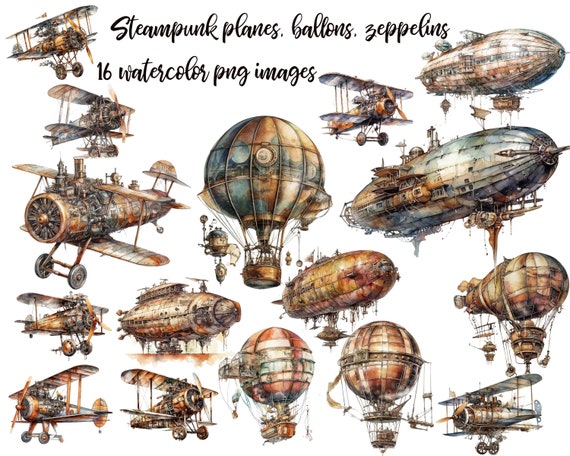The image showcases a collection of 16 steampunk-style watercolor illustrations of various aircrafts, including biplanes, hot air balloons, and zeppelins. The background is plain white, emphasizing the central elements without borders. At the top center, two lines of cursive black text read, "Steampunk Planes, Balloons, Zeppelins, 16 Watercolor PNG images." The illustrations are arranged with propeller planes predominantly on the left, hot air balloons in the center, and zeppelins mostly on the right. Each aircraft is characterized by a rusted, weathered appearance, painted in bronze-browns and greenish-blues, evoking a sense of aged metal. Notably, some hot air balloons integrate ship-like bodies or bases, enhancing their steampunk aesthetic.